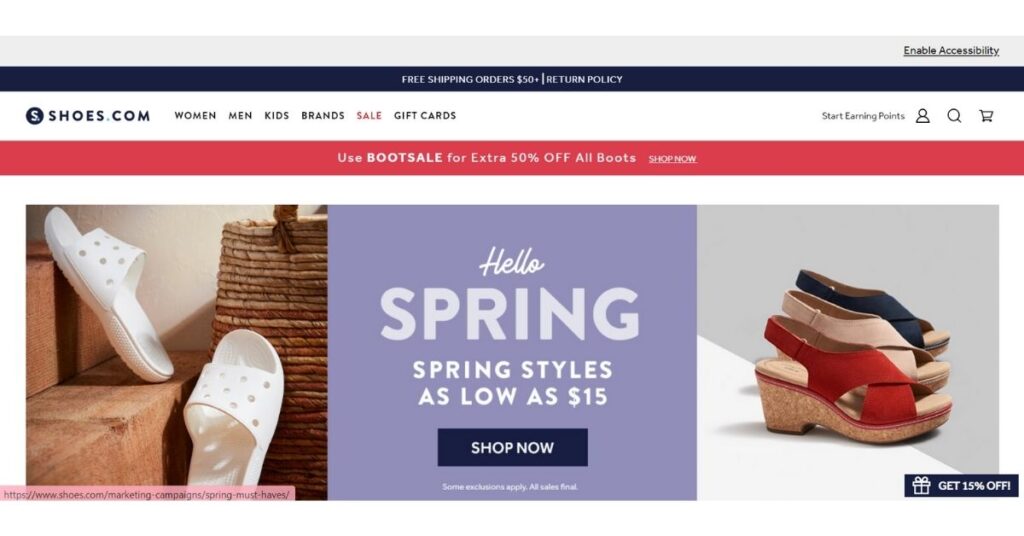This is an image of the homepage for the website shoes.com. The centerpiece of the page is dominated by the company's icon, a black circle featuring a white 'S' in the middle. The site serves a wide range of customers, offering shoes categorized for women, men, and kids, as well as a variety of brands. The navigation options are clearly laid out, allowing users to click on sections for sales, gift cards, or to use the search bar. Accessibility features are also enabled on the site.

At the top of the homepage is a large, eye-catching section predominantly hued in purple, with the welcoming phrase "Hello Spring" prominently displayed. This section highlights spring styles starting as low as $15 and includes a "Shop Now" button in black with white text for easy navigation.

The left side of this featured section showcases a pair of white women's sandals, artistically arranged on steps, with a basket placed behind the right foot. On the far right side, additional highlighted sandals in red, beige, and black are displayed on a floor divided diagonally into white and grey segments.

Above these images runs a striking red bar with a promotional message: "Use code BOOTSALE for an extra 50% off all boots," ensuring the sale offer is highly visible and easy to understand.